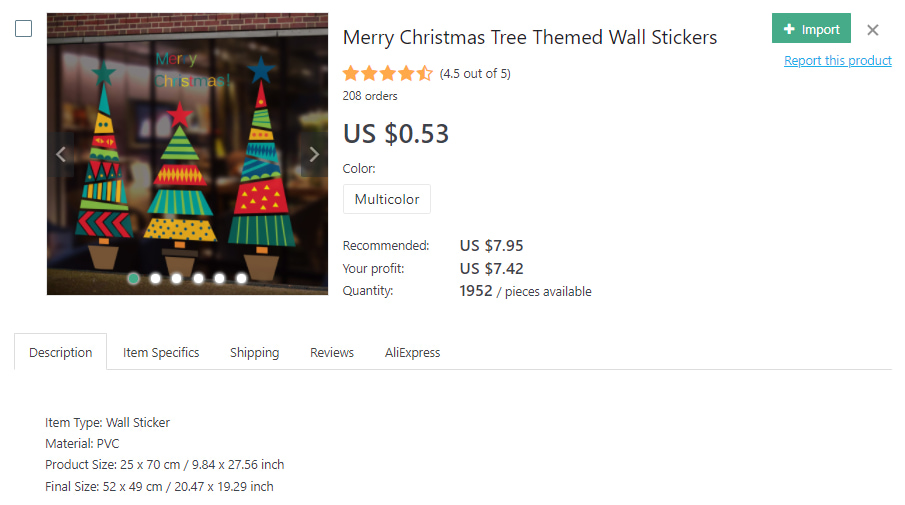This screenshot from an unknown website showcases a vibrant holiday-themed product. At the top left of the image, there is a photograph featuring a window adorned with three decorative Christmas tree decals. The leftmost tree is tall and cone-shaped, topped with a blue star, with its body composed of various geometric shapes in shades of blue, yellow, and red. The middle tree, bearing a red star atop, mirrors the style of the first tree. The rightmost tree similarly features a blue star, matching the others in design. Above the central tree, the phrase "Merry Christmas" is prominently displayed in alternating blue, red, yellow, and green letters.

To the right of the image, a text panel describes the product as "Merry Christmas tree themed wall stickers," noting that it is an imported item. The product has garnered a high rating of four and a half stars out of five from 208 orders and is priced at U.S. $0.53 per unit. The multicolor item promises a recommended retail price of U.S. $7.95, yielding a potential profit of U.S. $7.42 per piece.

Further details specify that 1952 pieces are available. The wall sticker is made from PVC material, with a product size of 25 by 70 centimeters (9.84 x 27.56 inches) and a final applied size of 52 by 49 centimeters (20.47 x 19.29 inches). Adjacent to the description are other menu options, including item specifics, shipping, reviews, and AliExpress.